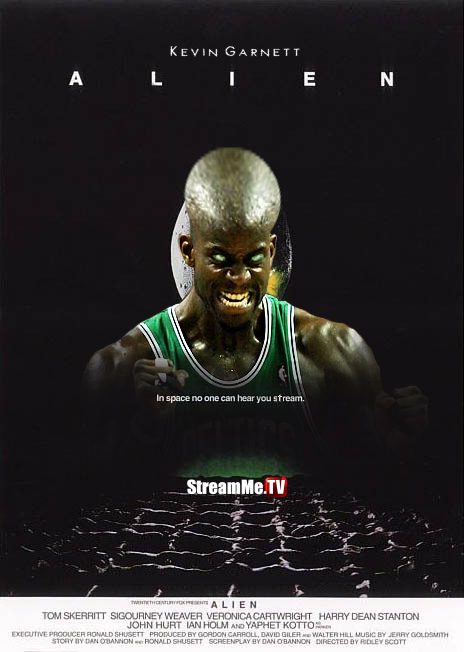The image is an advertisement for what appears to be a TV show or movie featuring Kevin Garnett transformed into an alien. The picture depicts the African-American basketball player in a green jersey, with his head morphed into an alien form. His eyes glow green, and his expression is a sinister scowl with gritted teeth, giving him a possessed look. Kevin’s head is unnaturally bulging and silver, further enhancing the alien appearance. His muscular shoulders are tensed, as if ready for action. 

The bottom of the image features a dark crisscross design, resembling theater seats or a heavy fishing net, adding to the eerie atmosphere. The caption underneath reads, "Kevin Garnett, alien. In space, no one can hear you stream," with a logo for streamme.tv. Below, there are credits listing "Alien" stars Tom Skerritt, Sigourney Weaver, Veronica Cartwright, Harry Dean Stanton, John Hurt, Ian Holm, and Yafit Koto. Additional credits include the executive producer, producers, musician, story writer, screenwriter, and director, suggesting this is a high-production value project.